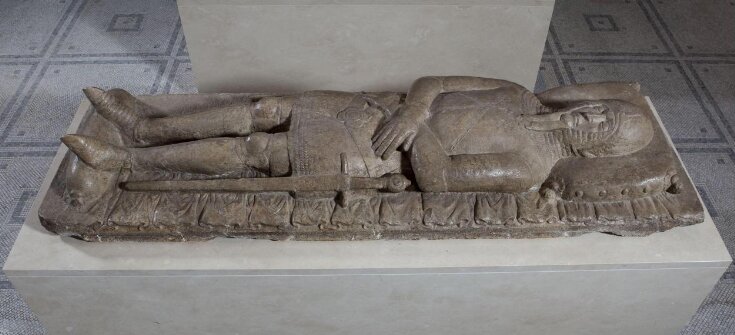The image depicts a medieval stone sarcophagus resting on patterned stone flooring, with a stone wall in the background. The sarcophagus is carved in great detail to resemble a medieval knight lying in repose. The knight's head rests on a pillow, and his eyes are closed, portraying a peaceful passing. He is depicted with chain mail and body armor, including a steel helmet atop mail that covers his head. His hands are folded over his stomach, and a sword is placed beside him, suggesting his warrior status. The knight's feet are adorned with pointed, jointed armor-plated shoes, and a bolster rests at his feet. This intricately carved stone structure captures the essence of a medieval soldier laid to rest, adorned in his battle attire.